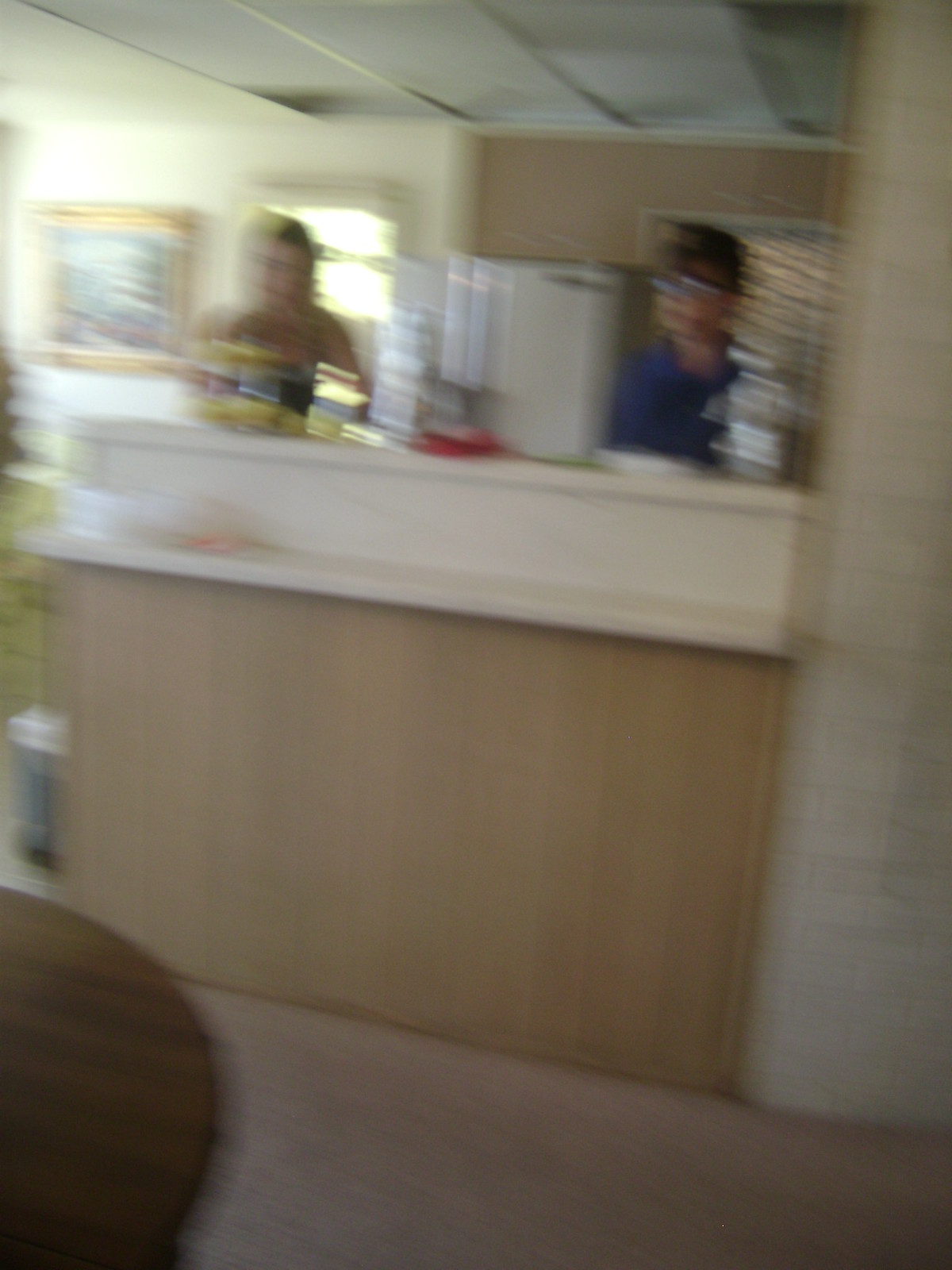A vertical, indoor photograph depicts a lively kitchen scene, albeit slightly blurred. The kitchen features a white drop ceiling and large window, allowing natural light to filter in. Dominating the foreground is a natural wood high countertop, adorned with various items. Behind the counter, two people are engaged in an activity, their forms indistinct but their presence adding a warm, bustling atmosphere. A white refrigerator stands in the background, near a wall adorned with a gold-framed picture. Just in front of the countertop, the corner of a dark wooden round table is visible, grounding the scene with a touch of rustic charm.